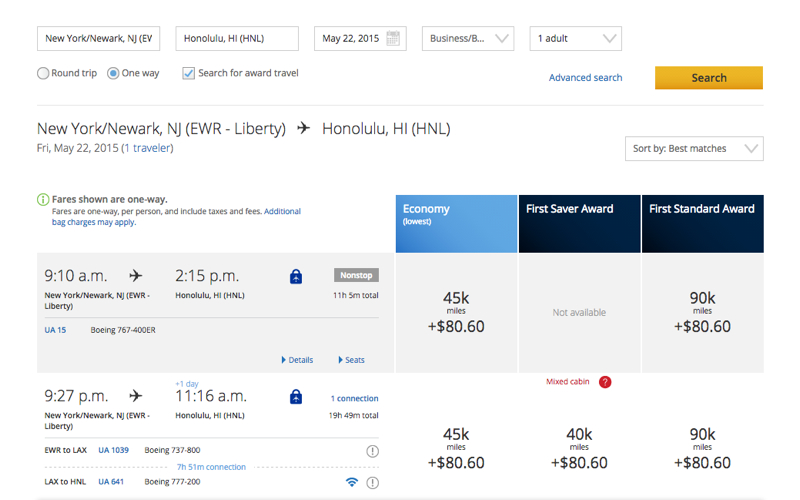This is a detailed view of a screenshot taken from a travel website, outlining the specifics for booking a flight:

At the top of the image, there's a white rectangular bar containing black text. It reads "New York/Newark, New Jersey (EWR)" followed by "Honolulu, Hawaii (HNL)." Next to this, it specifies "May" and directly underneath in a gray rectangle, the date "May 22nd, 2015" is displayed.

Further down, details about the trip are listed. It notes "BUSINESS/B," indicating the type of seating preference. This is followed by another dropdown in a rectangle showing "One Adult," confirming that a single traveler will be making the journey. Below this section, a clickable link in vibrant blue text reads "Advanced Search." Adjacent, a gold rectangle with white text says "Search."

The main details of the flight appear next. It specifies the route as "New York/Newark, New Jersey (EWR) - Liberty" to "Honolulu, Hawaii (HNL)." The flight date is reaffirmed as "Friday, May 22nd, 2015," with the notation "(One Traveler)" in cyan blue.

Moving down the page, there's a green circle housing an "i" symbol. Black text beneath it states "fares shown are one way," with lighter black text clarifying "fares are one way per person, and include taxes and fees," followed by a blue hyperlink indicating "additional bag charges may apply."

On the right side, several options are presented within rectangles. The first rectangle is cyan blue with white text that reads "Economy (Lowest)." Adjacent to it, in bold blue, are the options "First Saver Reward" and "First Standard Reward." 

The departure and arrival times are listed next. The first flight departs at 9:10 AM and arrives at 2:15 PM, traveling on a Boeing 767-400ER. Beneath this, another flight is shown departing at 9:27 PM and arriving at 11:68 AM (likely a typo for a realistic time).

Pricing and reward specifics are given:
- For "Economy" at 45k miles plus $80.60, "First Saver Reward" is not available.
- In "First Standard Reward," it is priced at 90k miles plus $80.60.
- Another flight in economy shows 45k miles plus $80.60.
- The "First Saver Reward" here is 40k miles plus $80.60.
- Lastly, "First Standard Reward" is set at 90k miles plus $80.60.

The detailed layout provides a comprehensive breakdown of pricing, available rewards, and flight times, helping travelers make informed decisions.